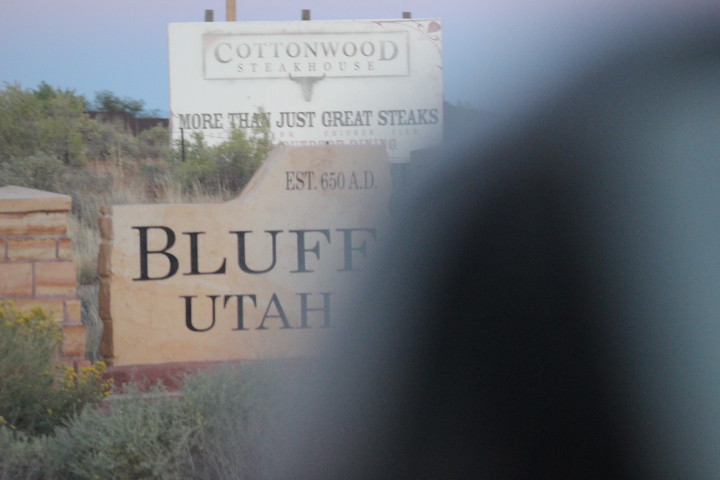The image depicts a somewhat obscure photograph, partially obscured by what appears to be a hand or finger covering the bottom right section with a dark, blueish shade. Central to the image, to the left, a significant, polished, light brownish stone is inscribed with red letters reading "Bluff, Utah," along with the establishment date "650 AD." Adjacent to this stone, there's a neatly cut reddish wall. Above the stone, a white sign supported by posts displays the name "Cottonwood Steakhouse" in black lettering, followed by the tagline "More than just great steaks." The background features a clear blue sky and verdant greenery, adding a touch of nature to the scene. Additionally, a blurred shoulder in possibly a gray or blue jacket appears in the foreground, suggesting accidental obstruction during the photo capture. The overall scene is framed with details such as scrub greenery and a decorative stone pillar on the left, enhancing the rustic and historical ambiance of the setting.